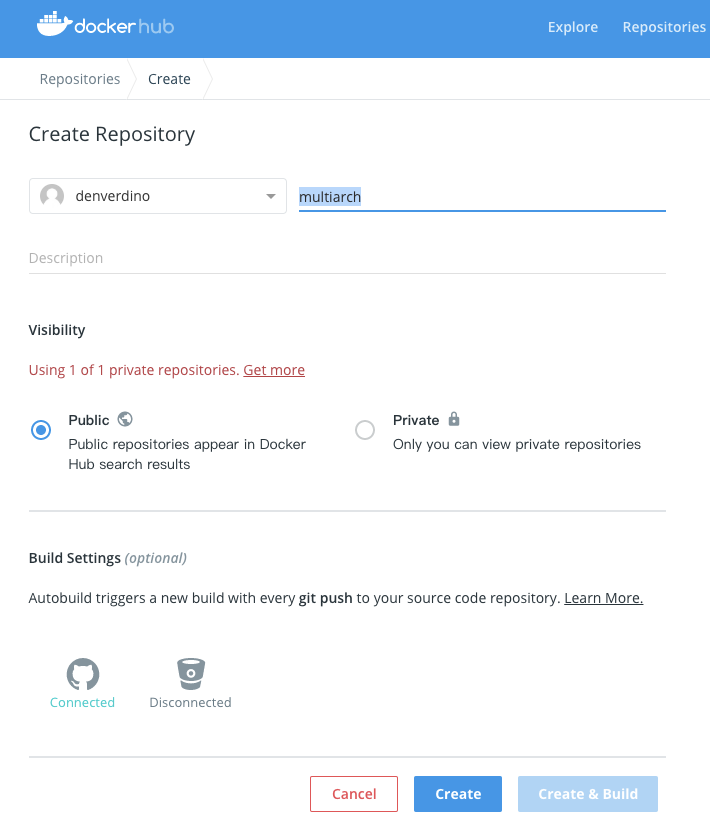Detailed Caption: 

This image is a screenshot from the Docker Hub website. At the top, there is a medium blue bar with a white whale logo that has box-like shapes on its back, symbolizing Docker’s logo. To the left, the bar displays the text "docker hub" in lowercase letters, with "docker" rendered in white and "hub" in a lighter blue.

On the right side of the top bar, the options "Explore" and "Repositories" are visible. The main body of the page is predominantly white. On the left, just below the main navigation bar, the options "Repositories" and "Create" are listed, separated by a light vertical line. Beneath this, the text "Create Repository" is shown.

A box beneath this area displays a user icon followed by the username "denver-dino." Next to it, "multiarch" is highlighted in blue over gray text, with a blue underline beneath it.

Further down on the left, the word "Description" is very faint with a subtle line below it, followed by the more bolded text "Visibility." It indicates "using one of one private repositories" with an additional prompt to "Get more" underlined and presented in red text.

Below the visibility section, there are two radio buttons. The left radio button, which is blue and selected, is labeled "Public" with a small globe icon next to it. Beneath "Public," it is noted that "public repositories appear in Docker Hub search results." The right radio button is labeled "Private" with an adjacent lock icon, specifying that "only you can view private repositories."

A horizontal line separates the sections, followed by the words "Build Settings" with "optional" in parentheses. A description underneath states "Auto build triggers a new build with every git push to your source code repository," with "Learn more" both capitalized and underlined. The term "git push" is displayed in a slightly darker font for emphasis.

The next identifiable section mentions "connected" in blue, with a gray circular icon next to it that resembles a cat's head. Adjacent to this icon is what looks like a small trash can labeled "disconnected" below it.

Towards the bottom right are three buttons. The "Cancel" button is styled with a red outline and red text. Next to it, a solid blue button with white text reads "Create." Finally, a lighter blue button features the text "Create and Build" in white.

This detailed layout illustrates the user interface and options available on a Docker Hub repository creation page.